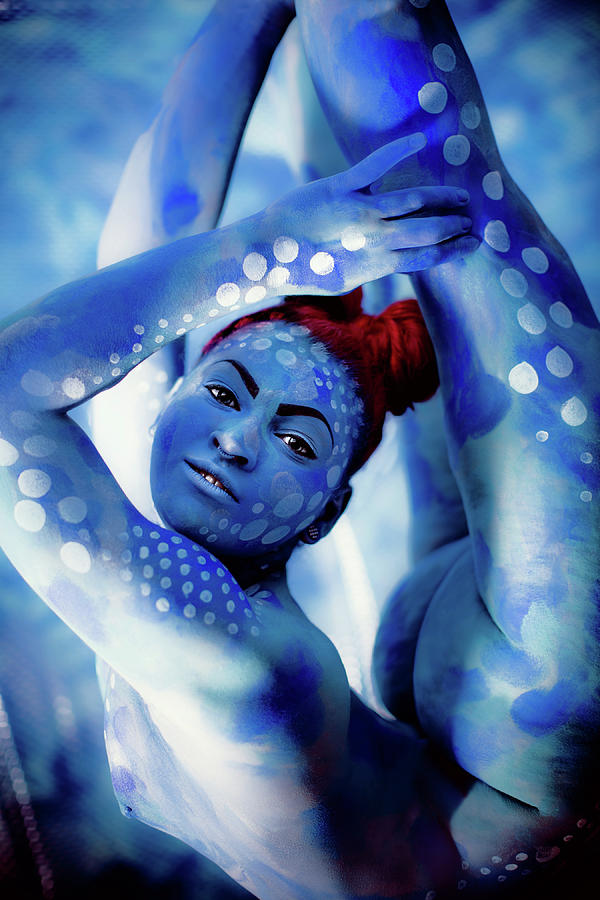This hyper-realistic image portrays a young woman engaged in a complex contortion pose reminiscent of yoga. The woman, completely naked, is covered in blue body paint adorned with white dots that resemble a starry night sky. Her vibrant red hair, styled into two buns, stands out against the monochromatic blue theme. She has a nose ring and pronounced dark eyebrows, adding to her striking appearance. Her body is twisted in such a way that she lies on her stomach while arching her torso and legs upwards, almost reaching over her head. She grasps her left knee with her left hand, displaying an incredible range of flexibility. Her face, framed by her colorful hair, gazes directly towards the camera, showcasing her dark eyes and white teeth. The background of the image is blurred and mirrors the blue hues and ethereal quality of her skin, enhancing the dreamlike atmosphere of the scene. The overall quality of the image is exceptionally high, emphasizing the intricate details and textures.